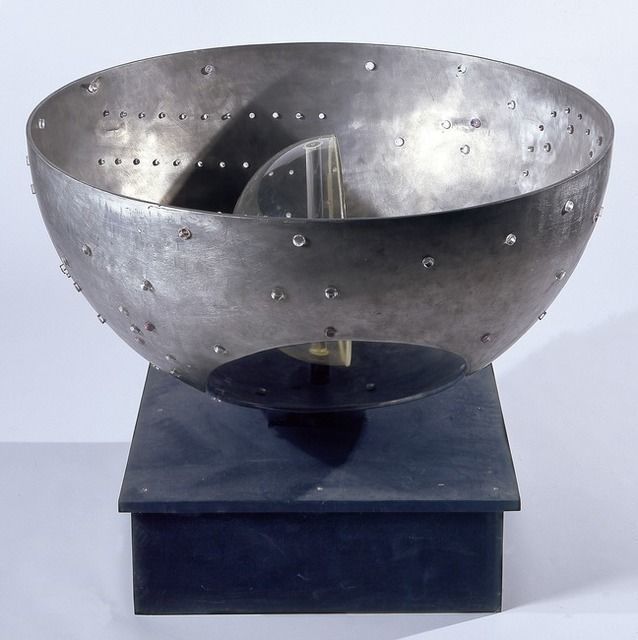The image depicts a meticulously arranged art display featuring a detailed composition of a silver metal bowl with numerous randomly-sized tiny holes, including a significant, perfectly circular hole at the front bottom taking up almost a quarter of the bowl's side. Inside this metal bowl stands another bowl on its side, made of clear glass with a slightly plastic appearance, and with yellow lines accentuating its rim. The entire arrangement is positioned on a blue stand, which resembles a rectangular box with a slightly larger top surface. The stand has a notable design with silver holes in each corner and another in the center, ensuring its stability on the white surface beneath. The background is a light gray, and the objects cast a pronounced shadow to the right, adding to the display's artistic intrigue.